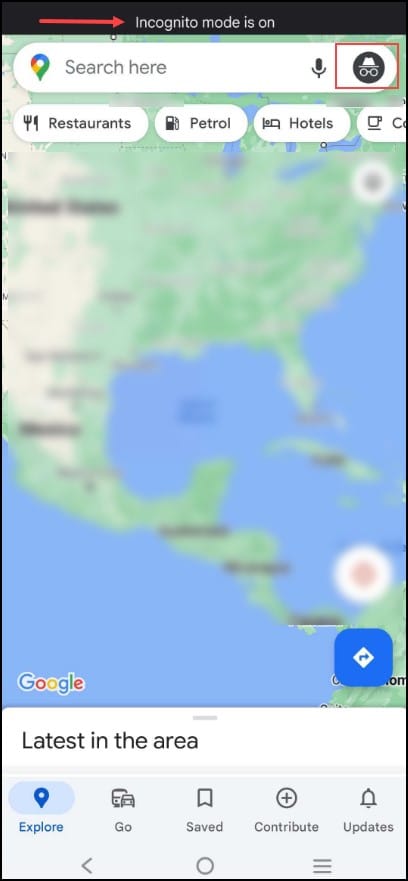This is a screenshot of a mobile phone displaying an incognito mode interface. At the top, a black bar runs horizontally across the screen with a prominent red arrow pointing to the middle of it. At the end of the arrow, white text reads "Incognito mode is on." Directly beneath this bar, there is a white search field. On the left side of the search field is a rainbow-colored location sharing symbol. In the center of the search field, greyed-out text reads "Search here." On the right side, there is a black microphone icon.

Additionally, there is a black circle with a white hat and glasses in the center, indicating incognito mode, which is highlighted by a red square around it. Below the search field, there are three buttons with white backgrounds and black text. The buttons are labeled "Restaurants," "Petrol," and "Hotels." 

Further down, there is a very blurry and out-of-focus map displaying the continental United States, Central America, Cuba, the Dominican Republic, and Haiti. The map appears to be censored. At the bottom of the screen, the word "Google" appears. Below this, within a white rectangle, there are several black text options: "Latest in the area," "Explore," "Go," "Save," "Contribute," and "Updates."